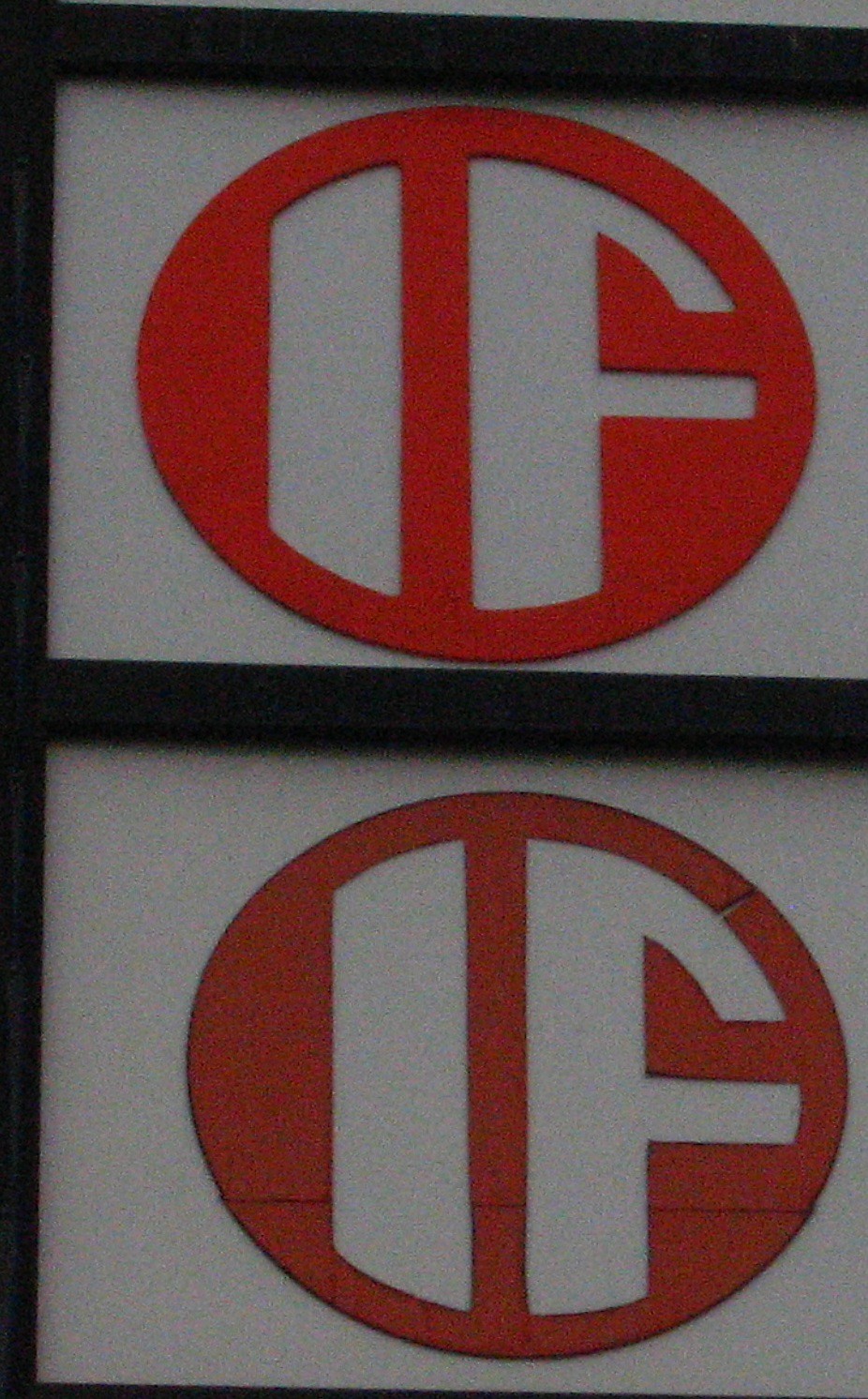This color photograph is divided into two sections, both set against a white background. Centrally placed in each section is an orange circular object, one above and one below. The upper part of the photograph features a neon orange circle, while the lower part displays a more muted, pale orange circle, indicative of age or wear. Each orange circle has cutouts in the shapes of the letters "I" and "F." A black metal frame horizontally bisects the photograph, creating a clear division between the two sections. The frame itself is cropped on the right edge, adding an element of incompleteness to the composition. The overall appearance of the lower section is more aged than the top, providing a visual contrast between the vibrant, neon upper circle and its faded counterpart below.